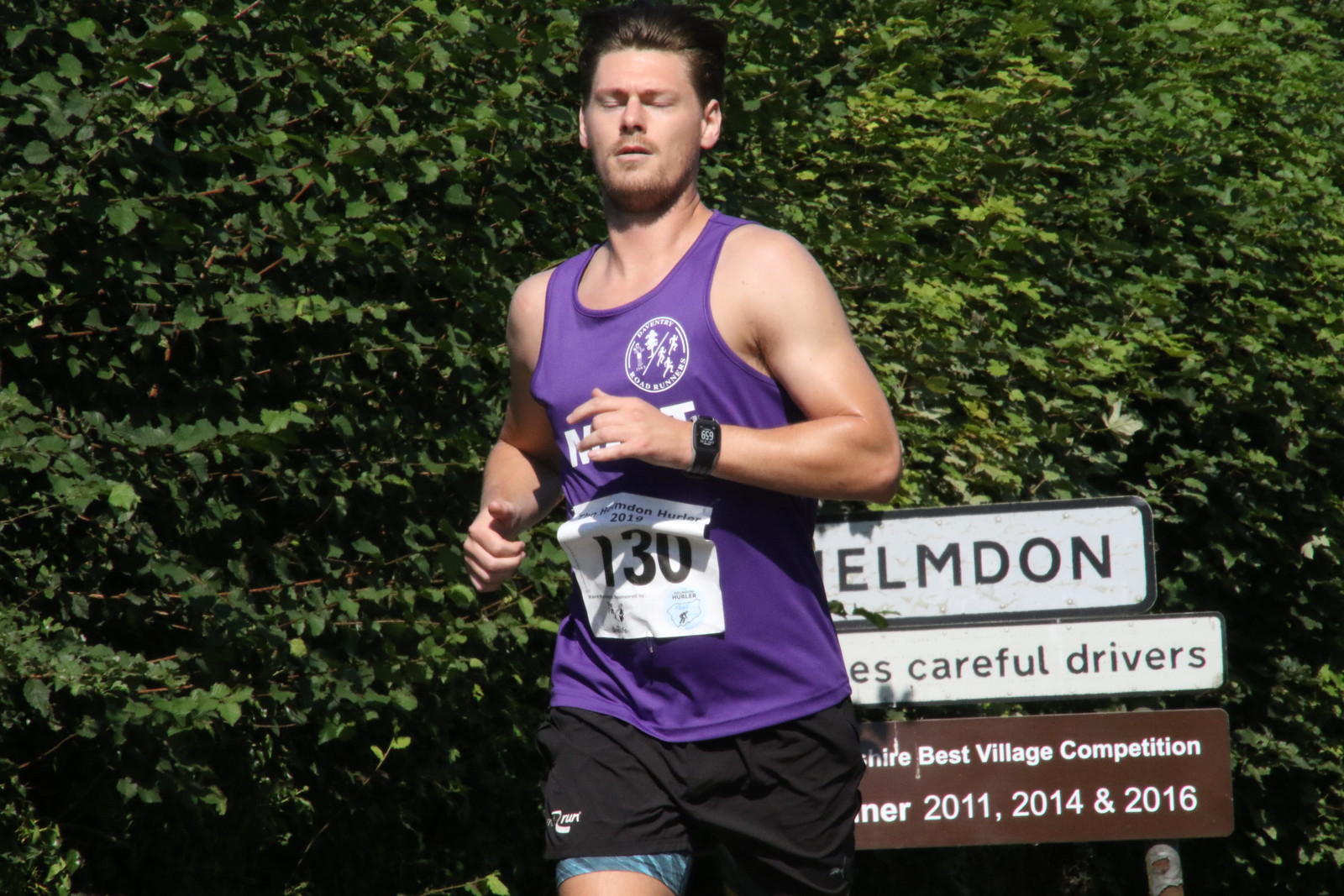In this image, a man is intensely running in a road race, donning a sleeveless purple jersey with the race number "130" prominently displayed on a white paper tag affixed to the front. He pairs this with black shorts, under which blue compression shorts are visible. He sports a wristwatch on his left wrist, and his eyes are closed as he runs forward. The background predominantly features lush green shrubbery, while a series of signs are partially obscured by the runner. The most visible sign, white with black letters, reads "ELMDON" and underneath it says "careful drivers," though the first word is obscured. Below this, a brown sign with white lettering announces accolades from the "Best Village Competition," specifically noting wins in 2011, 2014, and 2016. The runner's form and the vibrant outdoor setting underscore the intensity and focus of the moment.